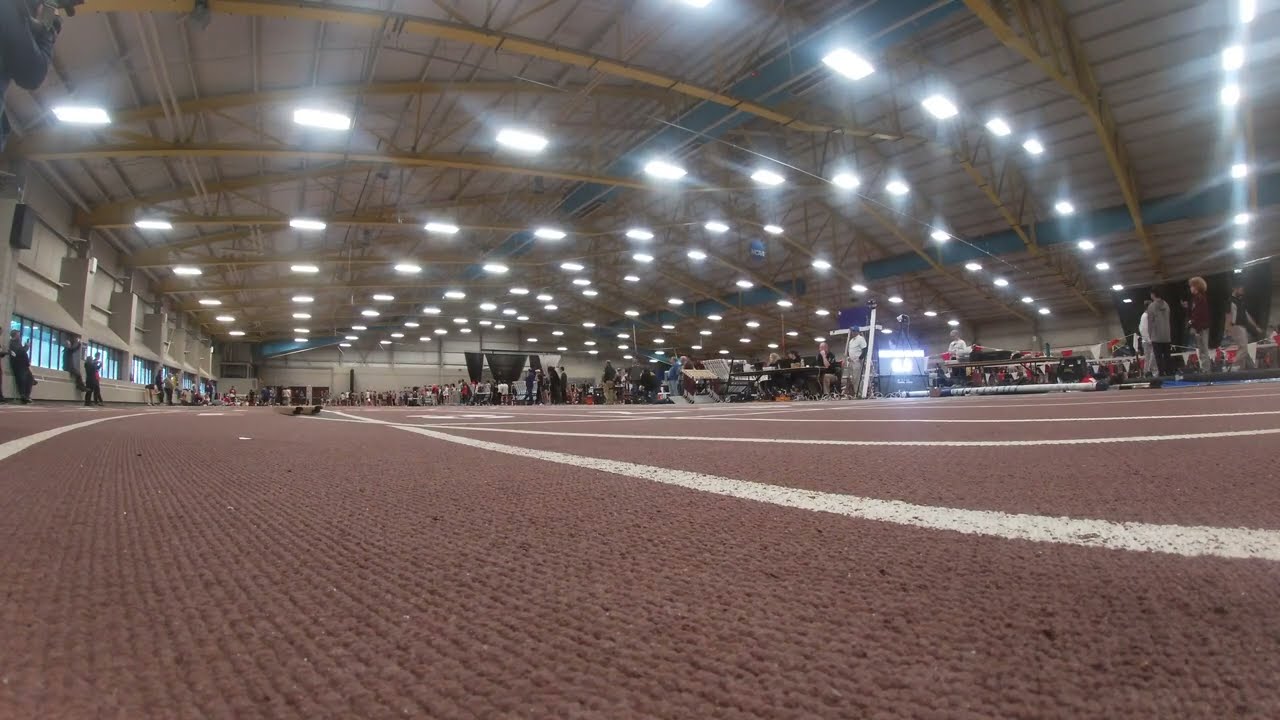The photograph captures a lively scene inside a vast event center, which resembles either a large gymnasium or an arena with high ceilings supported by steel beams and trusses. The image, taken from floor level, prominently shows the red carpeted floor with white painted stripes, likely designed for sports activities. Overhead, the ceiling is lined with numerous rows of lighting, brightly illuminating the spacious interior. 

The center is bustling with activity, with groups of people gathered around various booths and setups, suggesting an ongoing convention or expo. Some of the attendees appear to be vendors, possibly showcasing items related to hobbies such as video games, comic books, or collectibles. In the background, red and white pennants delineate specific areas, adding to the festive and organized atmosphere. The scene is filled with anticipation and preparation, as many people seem to be involved in setting up or waiting for participants, contributing to the dynamic and engaging environment of the event.